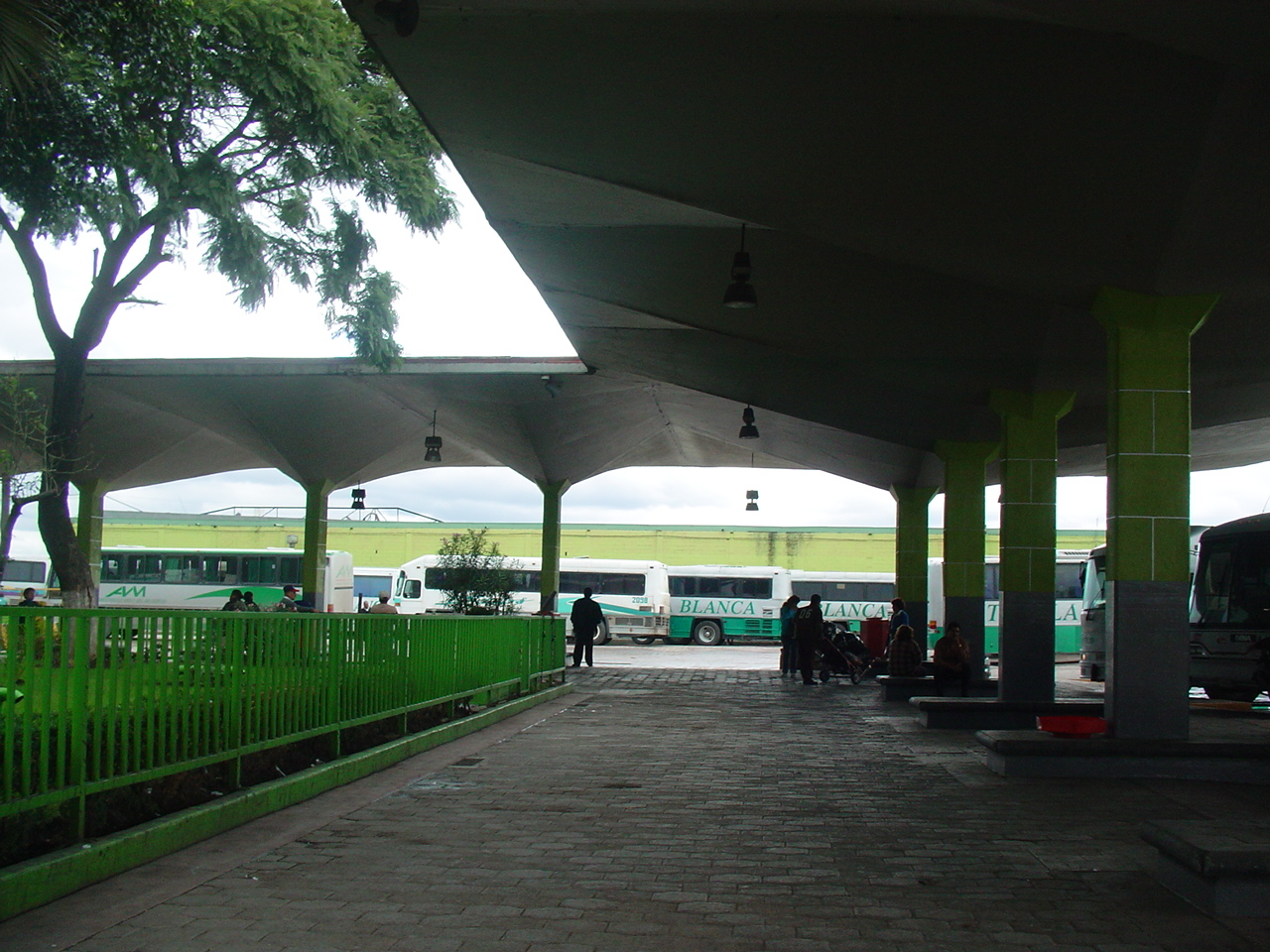The image captures an outdoor setting under a metal canopy that resembles a parking structure or bus depot, possibly linked to a tourist attraction. Multiple white and teal-green buses, prominently displaying the name "Blanca," are lined up underneath the canopy. To the right side of the frame, a bus with a slightly different design but similar colors has "AM" written on it. The structure is supported by four pillars with greenish-yellow tiles and concrete. On the left side, a green fence separates a grassy area with a tree, where a group of people is milling around, possibly congregating before boarding their buses. Light fixtures hang from the canopy, illuminating the brick-paved walkway underneath. The scene includes several individuals with luggage, suggesting they might be travelers awaiting transit, possibly from an airport or a hotel. Towards the center, a lone man stands with his back to the camera, facing the buses.